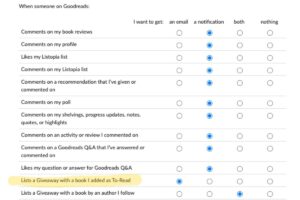This image, captured from a computer screen, depicts a section of a Goodreads notification settings page. The view is quite small, but it shows a list of different actions that can occur on Goodreads, such as "comments on my book reviews," "comments on my profile," "likes my listopia," "comments on my list," and "comments on a recommendation that I've given or commented on." Each action is listed on the left side of the page. The specific action "likes a giveaway with a book I added to read" is highlighted. To the right, there are four columns indicating the type of notifications the user can receive: "I want to get an email," "a notification," "both," and "nothing." The user has predominantly selected "a notification" for most actions, with specific preferences indicated for receiving an email about giveaways and both an email and notification for a particular action at the bottom of the list.